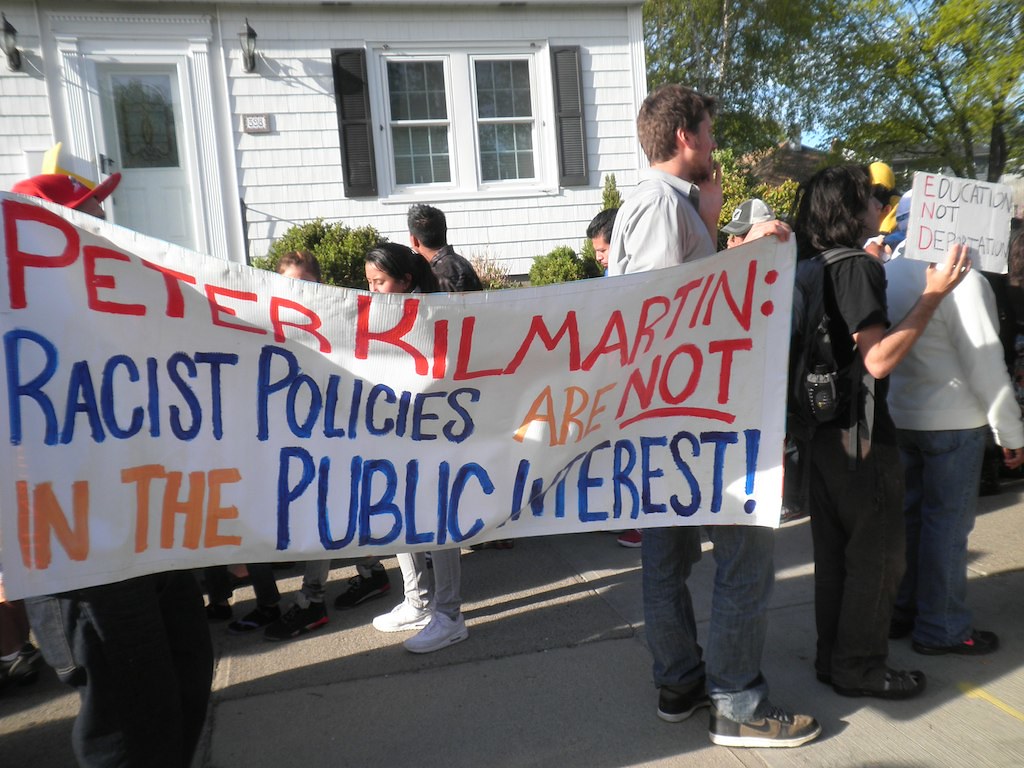In this horizontal rectangular image taken outside on a street or sidewalk, several people are participating in a protest. The backdrop features a white painted house with black shutters, a white front door topped with a window, and two visible windows on the front facade. To the right of the house, there are green trees and bushes.

A group of mostly younger individuals, dressed casually in jeans and a mix of short- and long-sleeve shirts, is gathered, seemingly marching or walking. They are predominantly facing towards the right. 

Prominently displayed in the center-left is a large white banner held by a few protesters. The text on the banner boldly addresses "Peter Kilmartin" in red, followed by the phrase "racist policies are not in the public interest." The intricate color scheme of the text includes red for "Peter Kilmartin" and "not," orange for "are," and blue for "racist policies" and "public interest."

Toward the right side of the image, another woman dressed in black holds a smaller sign that reads, "Education not deportation," with the first letter of each word in red, spelling out "END." The crowd mostly looks youthful, and while many of their faces are not fully visible as they gaze in different directions or are obscured by the banner, their collective stance is one of unity and protest.